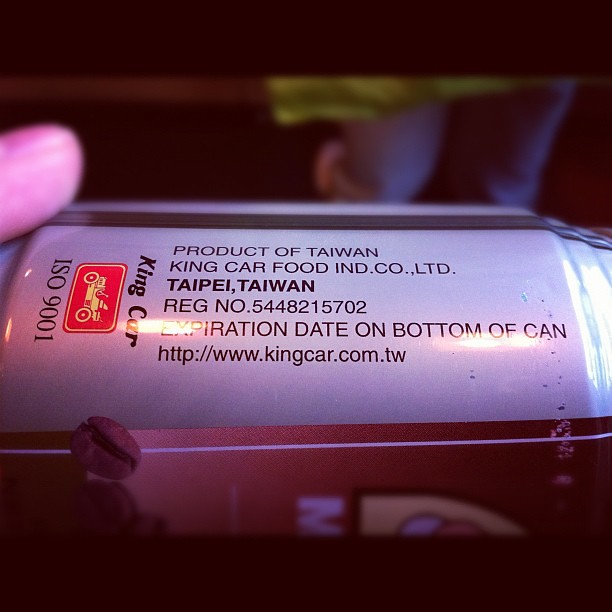A close-up image of a drink can being held sideways in someone's left hand. The can, shorter than usual, is predominantly a brownish-red or burgundy color and has a reflection of light on it. It features detailed black lettering on a lighter mauve background, prominently indicating its origin as Taipei, Taiwan. Below the main text, a red label with the brand name "King Car" is visible. The background of the photo is not well-lit, focusing attention primarily on the can.